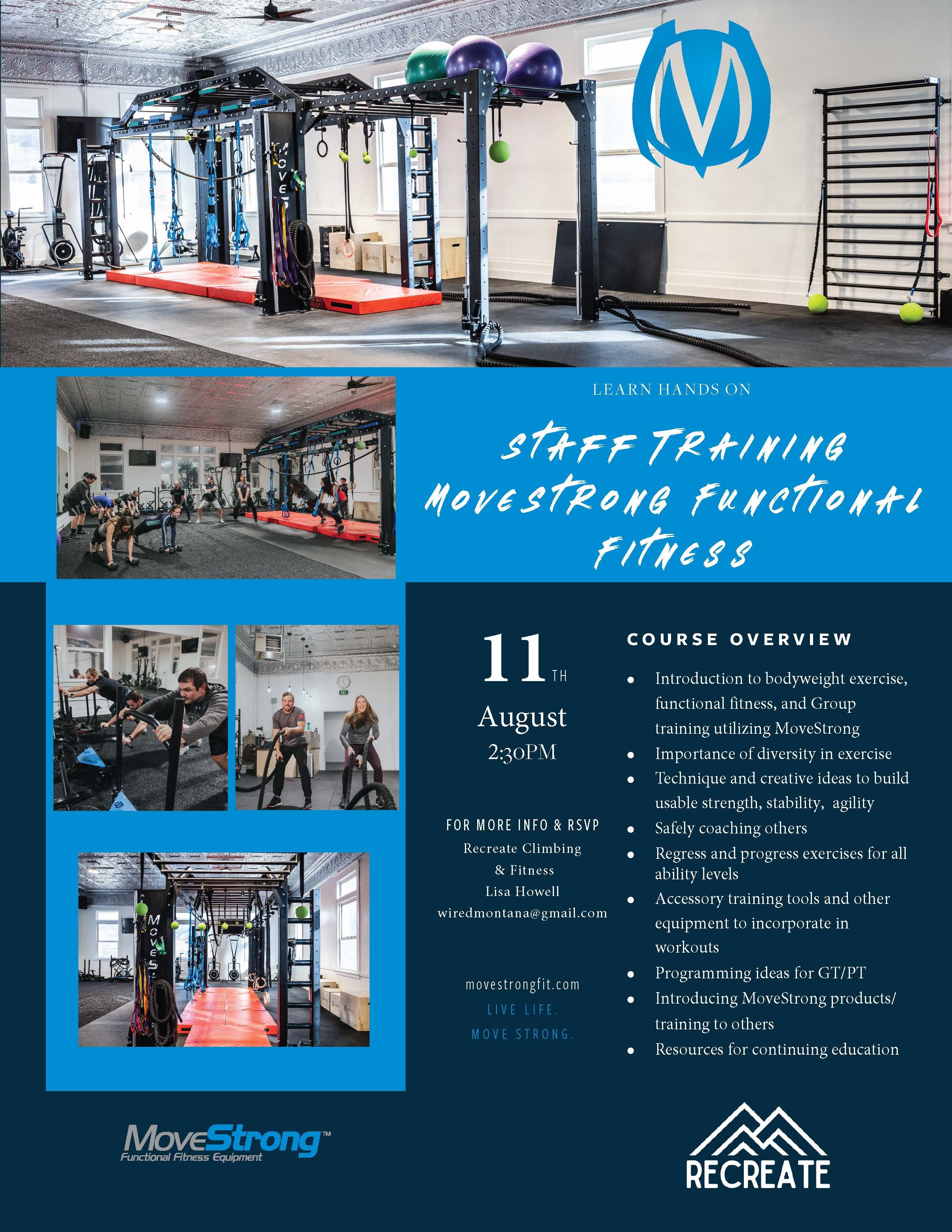This detailed promotional flyer for a staff training course on functional fitness, titled "Move Strong Functional Fitness," is set against a navy and light blue background, accented with colors like white, black, red, gray, purple, and green. The main image, occupying the top 25-30% of the flyer, showcases an empty gym, which appears to be in a warehouse setting, filled with elements like monkey bars, swinging ropes, yoga balls, mats, and elliptical machines. In the bottom left corner, three smaller, vertically-stacked photos depict people engaging in various workouts such as push-ups over weights and exercises on the monkey bars.

The central section features a light blue column with more images of people using gym equipment, accompanied by handwritten white text reading "Learn Hands-On Staff Training Move Strong Functional Fitness." The right side details the event information: "August 11th, 2:30 p.m." with instructions to RSVP to Recreate Climbing and Fitness through Lisa Howell (contact: wiredmontana@gmail.com). Below this, a course overview lists topics such as introduction to bodyweight exercises, functional fitness, group training, safe coaching techniques, and the use of Move Strong products and equipment.

At the bottom, the flyer includes the logos of "Move Strong" in gray and blue on the left, and "Recreate" in white on a dark blue background on the right.